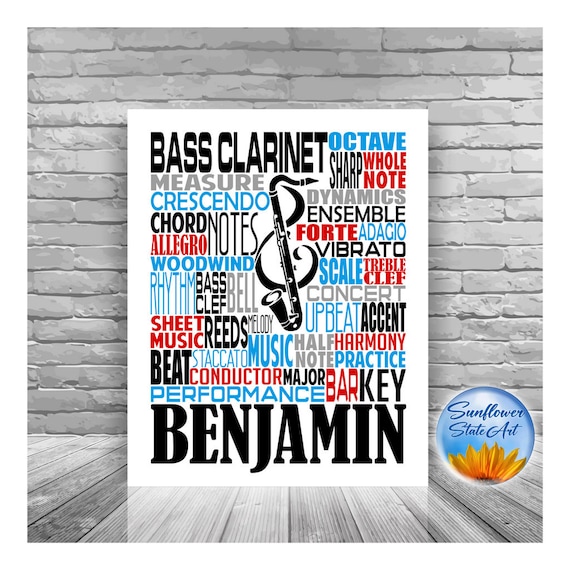The digital image showcases a rectangular sign leaning against a gray brick wall, with a light gray wooden floor beneath it. The sign, primarily focused on the theme of playing bass clarinet, features a variety of music-related terms in black, light gray, blue, and red text. Words such as "bass clarinet," "octave," "sharp," "whole note," "dynamic," "measure," "crescendo," "ensemble," "chord," "allegro," "notes," "forte," "adagio," "vibrato," "woodwind," "scale," "treble clef," "rhythm," "bass clef," "bell," "concert," "upbeat," "accent," "sheet music," "reeds," "melody," "music," "half note," "harmony," "practice," "staccato," "beat," "conductor," "major," "bar," "key," and "performance" are interspersed across the sign. Dominating the bottom portion is the name "Benjamin" in large print. Centrally placed on the sign is an image of a clarinet with a saxophone mouthpiece, superimposed on a treble clef. To the right of the sign, a small, colorful button featuring the text "Sunflower State Art" alongside a sunflower adds a distinct touch to the scene.